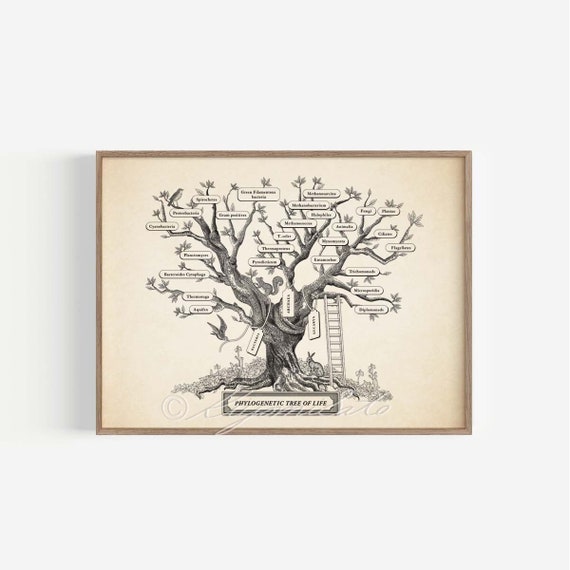This framed black and white illustration, set against an off-white, aged paper, depicts the Phylogenetic Tree of Life. Enclosed in a medium-toned brown wooden frame, the piece features a tree with a thick trunk and sprawling roots, which eventually splits into multiple trunks. The intricate branches and leaf springs are adorned with white rectangular or oval tags signifying different branches of the phylogenetic tree, though the labels are too small to read clearly. A ladder rests against the tree, and at its base, grass, a couple of birds, and a rabbit add life to the scene. Below the illustration, a banner inscribed with "Phylogenetic Tree of Life" is displayed, with a barely visible copyright watermark beneath it. The bottom of the illustration carries some barely discernible white script letters which seem to indicate the creator's name, though it remains unreadable. The entire artwork is against a simple white wall backdrop.